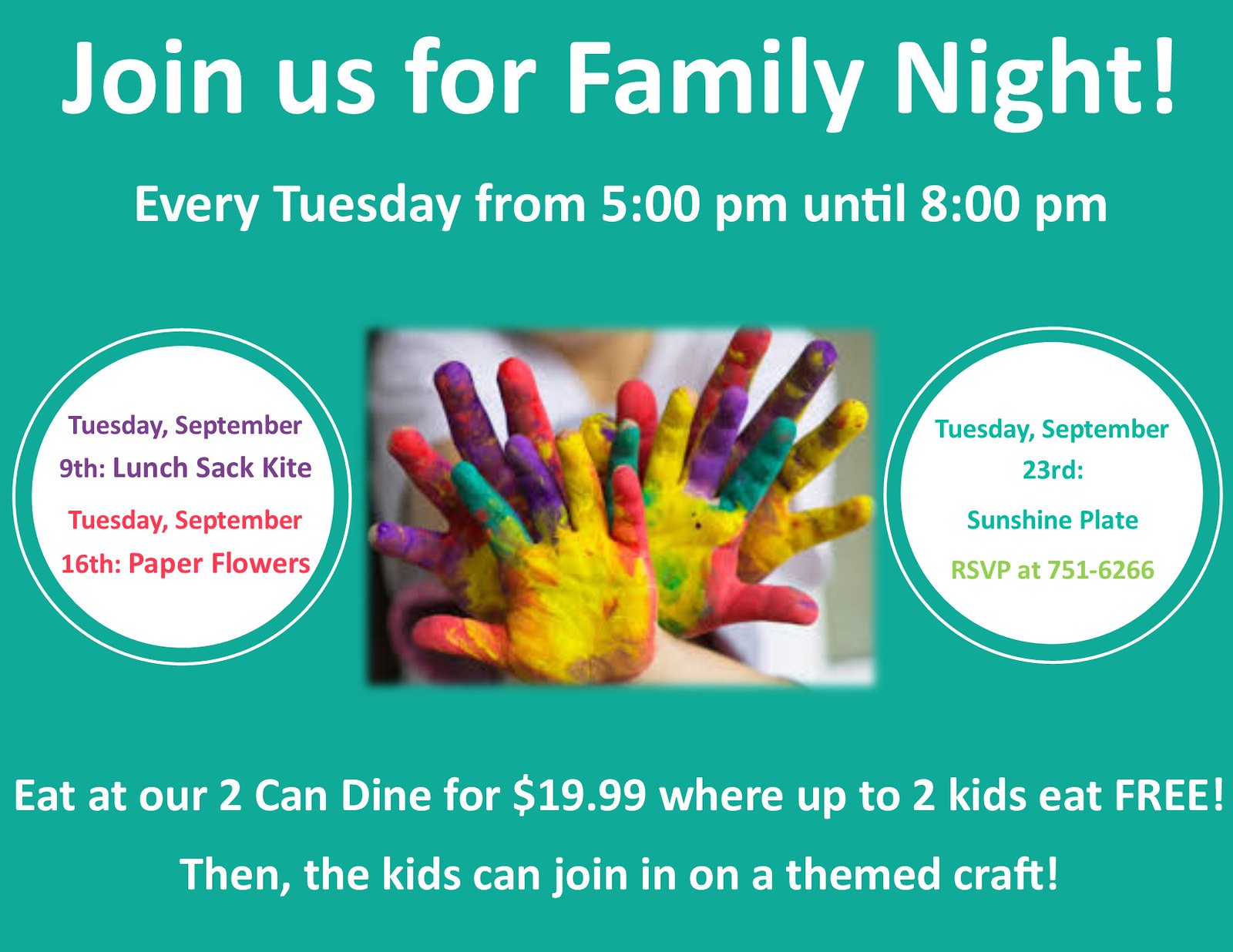This poster, set against a teal background, invites families to join for Family Night. At the top, white text proclaims "Join us for Family Night!" followed by subtext that reads "Every Tuesday from 5 p.m. until 8 p.m." Central to the poster is a vibrant image of children's hands painted in an array of colors—green, yellow, red, and purple—gathered together, with a person in a hazy white v-neck shirt in the background.

To the left of the image, inside a white circle, purple-blue text states the activities: "Tuesday, September 9th: Lunch Sack Kite" and "Tuesday, September 16th: Paper Flowers." On the right, another white circle features turquoise text detailing "Tuesday, September 23rd: Sunshine Plate," and provides an RSVP number: 751-6266.

At the bottom, the poster highlights a dining deal in white text: "Eat at our Two Can Dine for $19.99, where up to two kids eat free. Then the kids can join in on a themed craft."